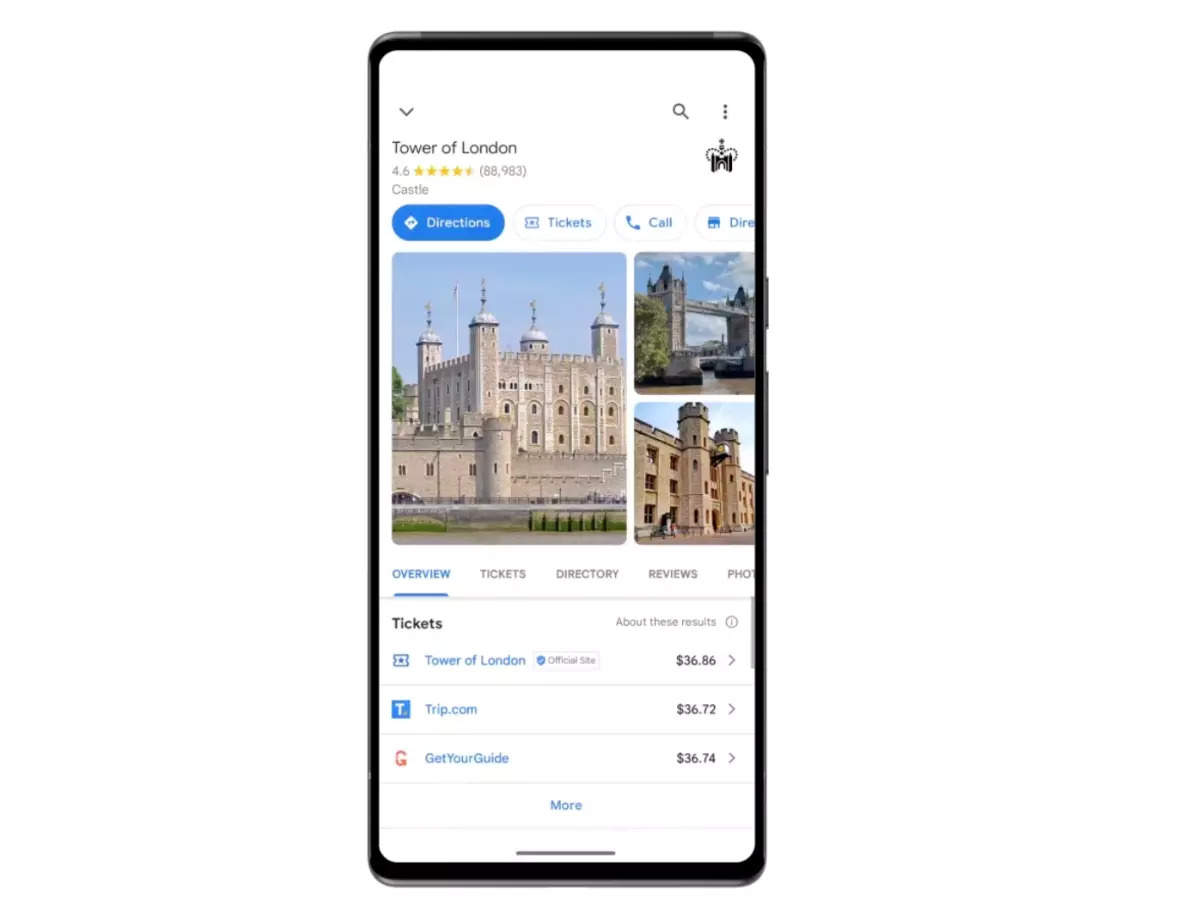A detailed screenshot image of a mobile phone interface presents information about the Tower of London. The phone screen, encapsulated in a black frame, allows visibility of two buttons located on the right-hand side, confirming that the entire phone, not just the display, is captured. The display itself features a clean, white background with rounded corners. At the top is a down caret pointed at the "Tower of London," rated with 4.6 stars by 88,983 reviewers under the category "Castle."

The interface contains a navigation bar with selectable tabs such as "Directions," "Tickets," and "Call," with "Directions" being currently highlighted. Just below, a prominent image of the Tower of London appears on the left, flanked by two smaller images on its right.

Further down, the screen presents options including "Overview," "Tickets," "Directory," "Reviews," and "Photos," with the "Overview" tab actively selected. Ticket prices are displayed next; the official Tower of London site lists a ticket price of $36.86, while competitor prices include $36.72 from trip.com and $36.74 from GetYourGuide—indicating slight variations but overall comparable rates.

This screenshot highlights key elements and pricing information, suggesting that the user is exploring or planning a visit to the historic Tower of London.